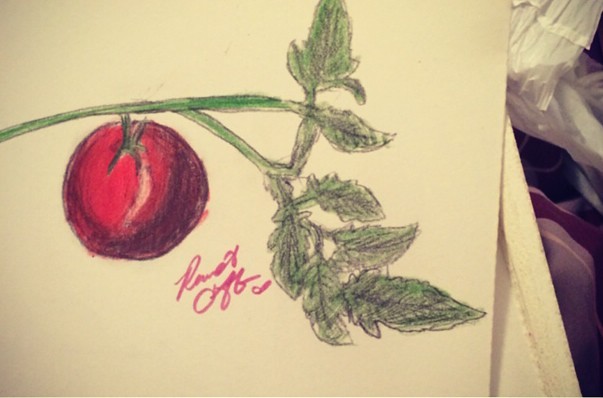This photograph features an amateur drawing on a sheet of white paper, though due to the lighting, the paper appears to have a sepia yellow hue. The drawing depicts a vibrant, red tomato hanging from a green vine, which extends outward with several leaves. The setting seems to be an informal living space, evidenced by the corner of a plastic bag visible in the background to the right of the image. The artist has signed the work with an initial "R," although the signature is somewhat difficult to decipher. The overall composition suggests a casual, home setting and a budding artist capturing the simple beauty of nature.